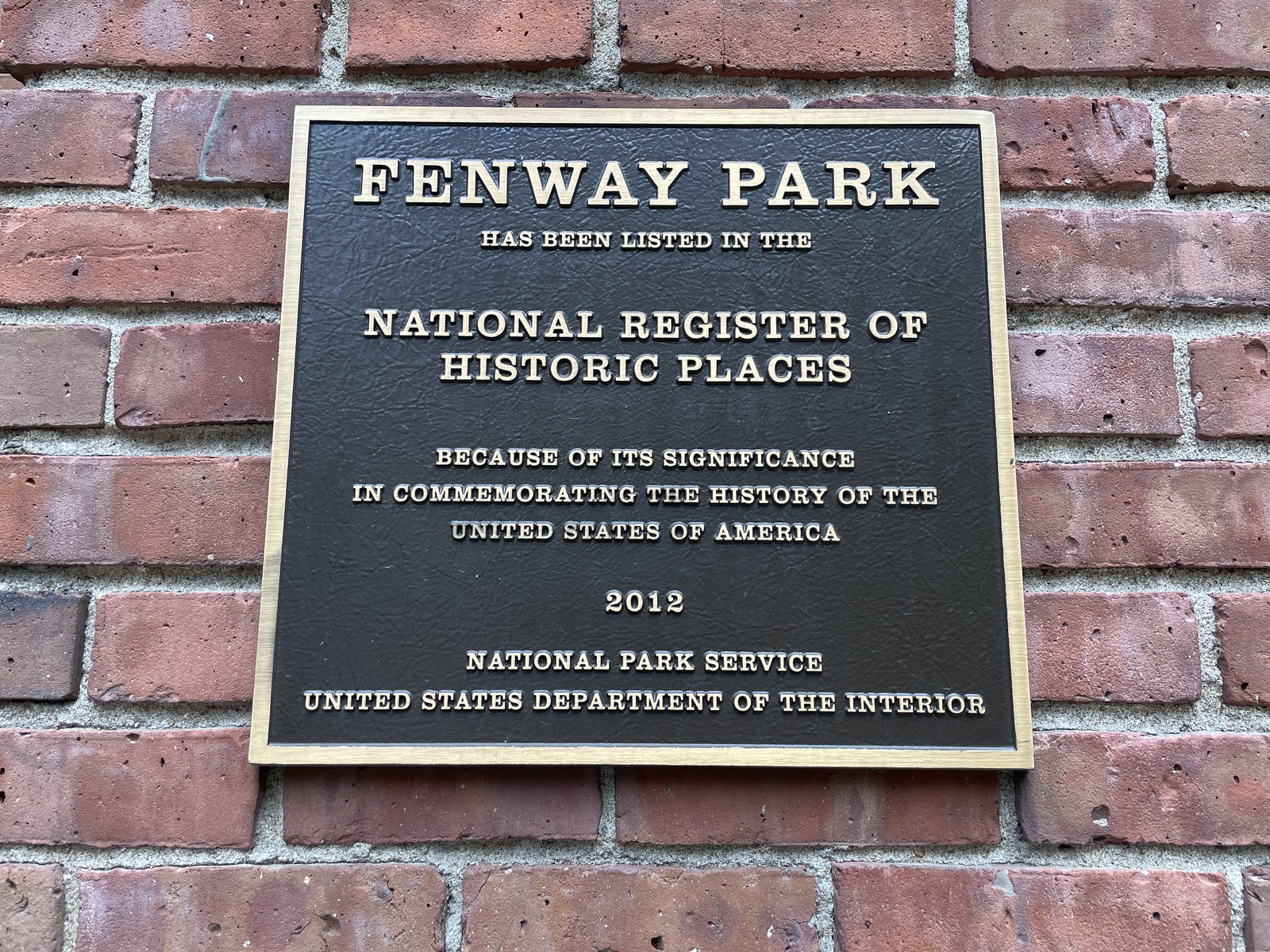This is a photograph of a plaque on a red brick wall, recognized for its historical significance. The plaque is black with gold borders and lettering, stating: "Fenway Park has been listed in the National Register of Historic Places because of its significance in commemorating the history of the United States of America, 2012. National Park Service, United States Department of the Interior." This gold and black placard is prominently positioned in the center of the image on the well-preserved, multi-toned red brick wall with white caulking, underscoring its importance and well-maintained condition. The plaque's clear and large text makes it easy to read and stands out against the crisp, undamaged backdrop of the bricks, accentuating the historic nature of Fenway Park.